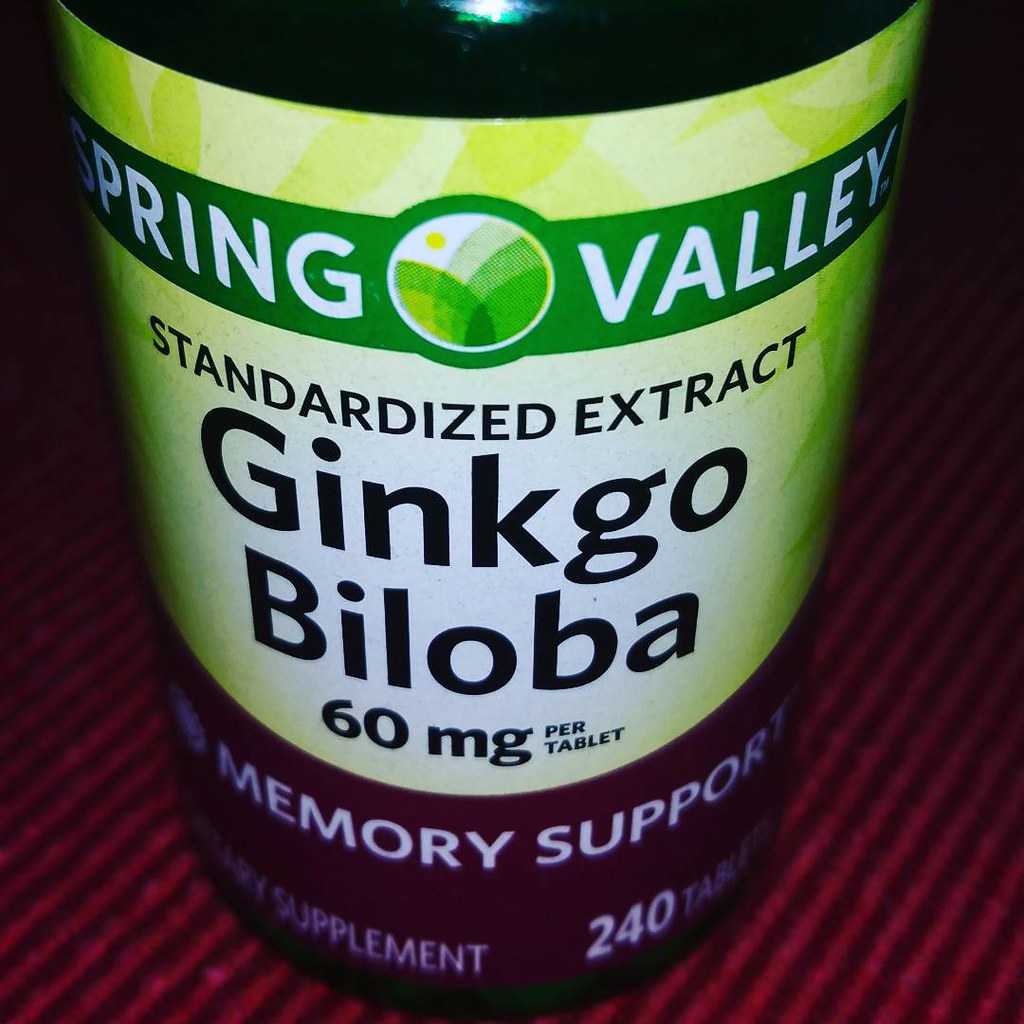The image showcases a supplement bottle placed on a dark red and light red striped tablecloth. The bottle features a yellow, green, and white label from the brand Spring Valley. The brand name, "Spring Valley," is written in white text on a green background, with a logo situated between the words "Spring" and "Valley." The logo is a circle with a white background, displaying several shades of green and a small, curved yellow sun. Below the brand name, in black text, it reads "Standardized Extract," followed by "Ginkgo," and "Biloba," both also in black. The dosage "60 mg per tablet" is clearly indicated. The label further states in white text "Memory Support," and at the bottom, it specifies "Dietary Supplement," and contains "240 tablets."